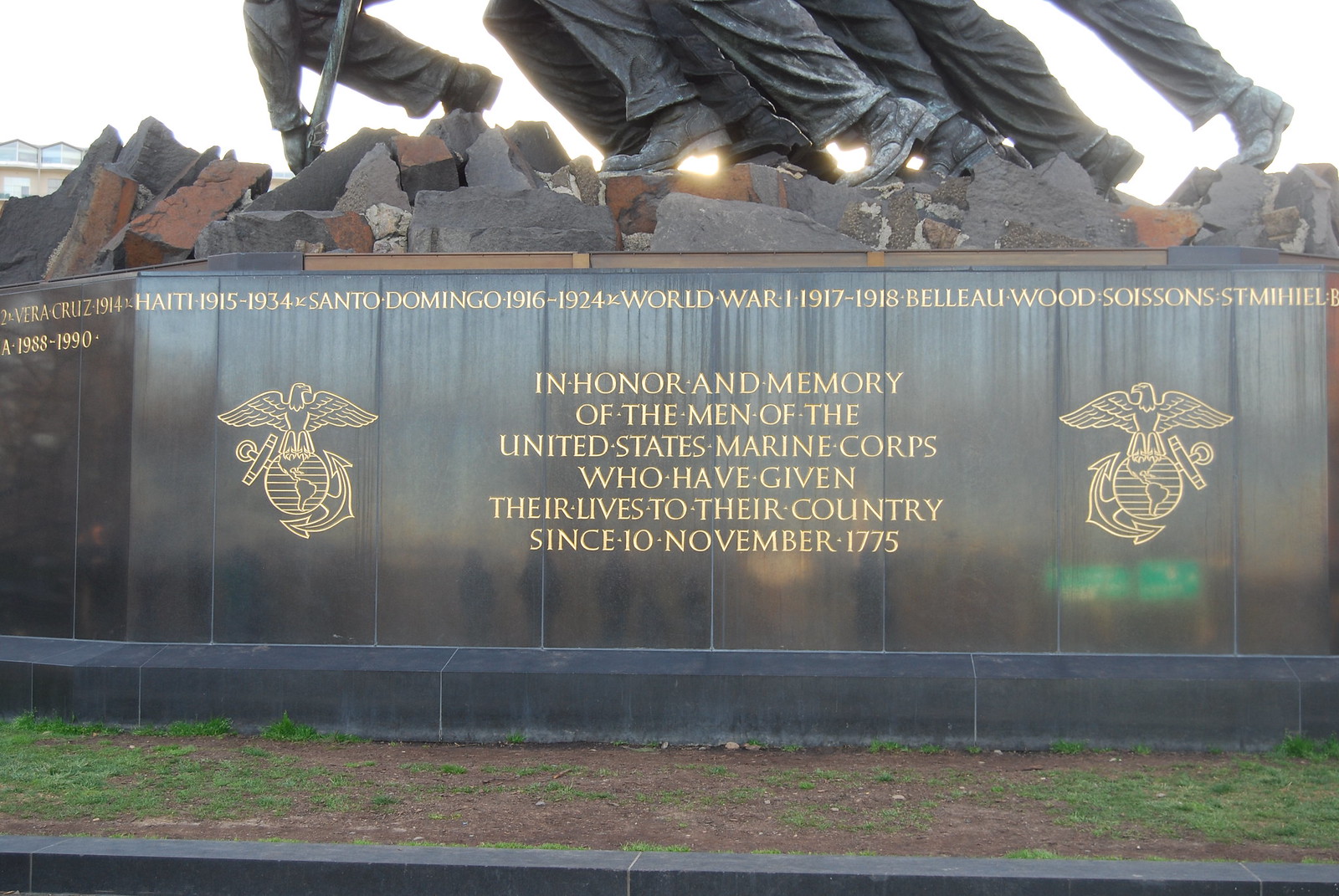The photograph is a color outdoor image capturing the base of a monument dedicated to the United States Marine Corps. The monument's base is composed of black stone with engraved gold text detailing significant historical battles and wars, such as Veracruz 1914, Haiti 1915 and 1934, Santo Domingo 1916 and 1924, World War I 1917 and 1918, Belleau Wood, Soissons, San Miguel, and extending to 1988-1990. Prominently, there is a tribute message in the center reading, "In honor and memory of the men of the United States Marine Corps who have given their lives to their country since 10 November 1775." Flanking this message are two gold Marine Corps emblems featuring an eagle perched atop a globe with an anchor in the background. The visible part of the statue above the base shows the legs and boots of Marine figures. The scene is set outdoors on a patch of ground with grass and dirt, bordered by a black curb, emphasizing the monument's solemn presence.